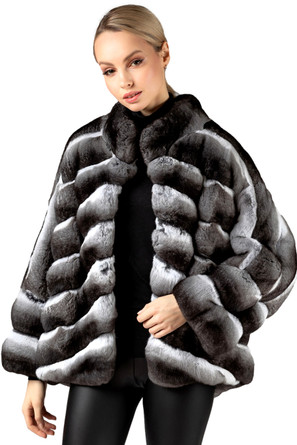This image features a striking portrait of a Caucasian model in her early twenties, standing against a stark white background with no other visible elements. The focus is on her chic ensemble, led by an oversized fur coat that combines luxurious materials and contrasting tones. The coat boasts a fluffy black collar and textured gray sections that cascade from the shoulders down to the arms, suggesting a cross-season fashion piece. Beneath the open coat, she sports a sleek black shirt paired with black leather pants, adding a sharp, edgy element to the look.

The model's dirty blonde hair is pulled back into a sleek ponytail that highlights her fair skin and subtle makeup, including light lipstick. Her direct, yet slightly tilted head angle and soft, sly smile give her a poised and sophisticated demeanor. Her left hand clutches the bottom part of her coat, casually opening it up to reveal the outfit beneath, while her right arm hangs straight by her side. This meticulous composition and the model's confident posture evoke the stylized elegance often seen in high-end fashion magazines.